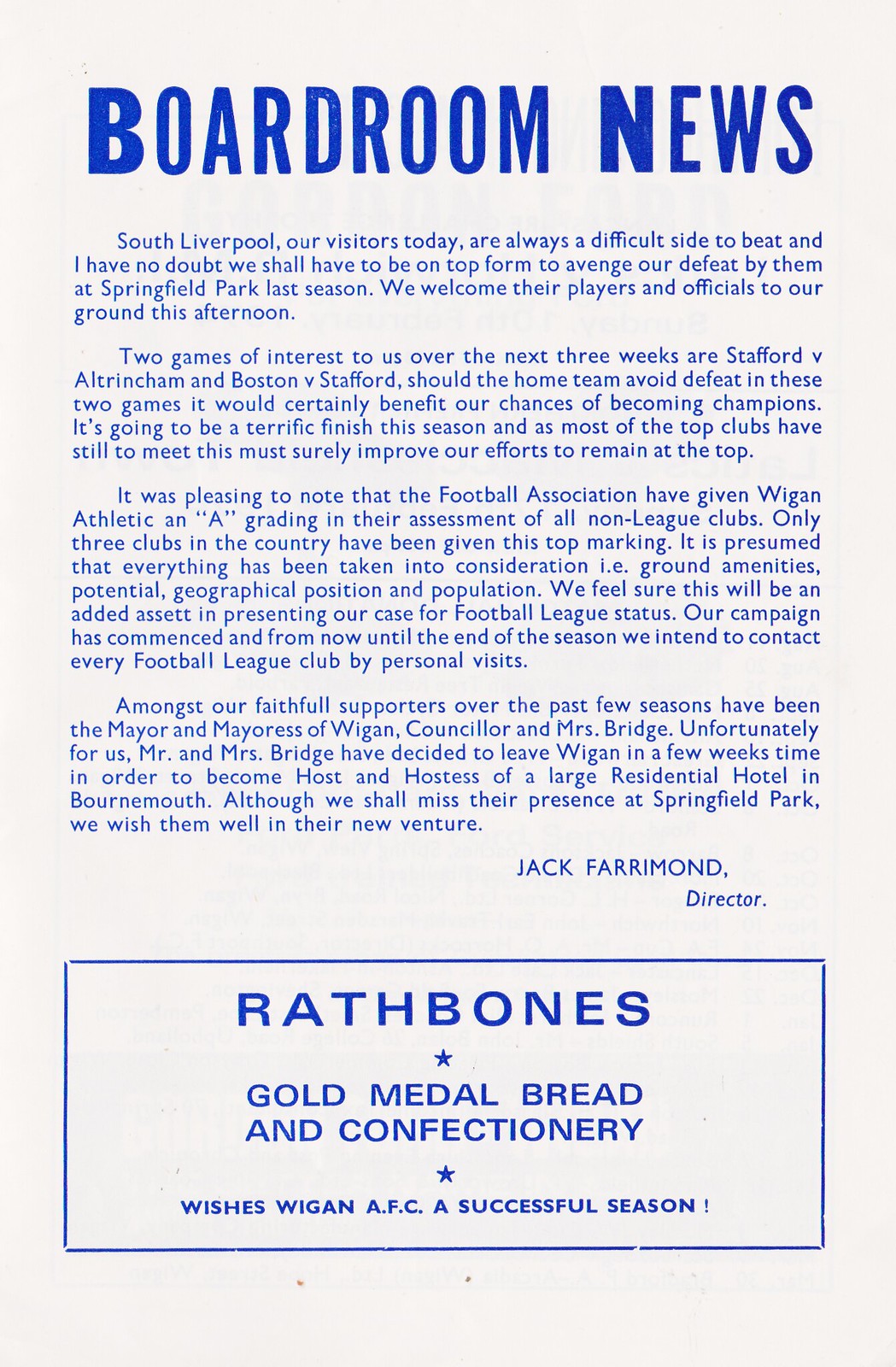The image in question is a single-page print on white stock, resembling a newsletter or insert from a magazine, likely intended to be a poster. The entire print uses blue ink, creating a cohesive look. At the very top, in large, bold, all-caps letters, it prominently reads "BOARDROOM NEWS." 

The main content of the text, which resembles a formal announcement or note, is written by Jack Faramond, the director. In smaller blue text, it states: "South Liverpool, our visitors today, are always a difficult side to beat, and I have no doubt we shall be on top form to avenge our defeat by them at Springfield Park last season. We welcome their players and officials to our ground this afternoon." 

Below this message, encased in a blue outline but set against the same white background, is another announcement: "Rathbones. Gold Medal Bread and Confectionary. Wishes Wigan AFC a successful season." The page does not contain any additional content, making these points the central focus.